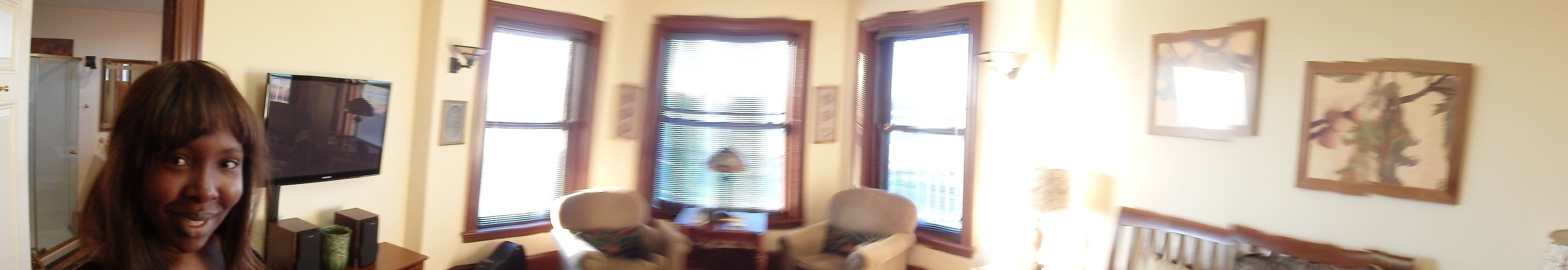In this vertically oriented photograph, we glimpse an interior corner of a home. A Black woman with light brown hair appears in the left corner of the image, captured from the neck up. Behind and slightly to her right, a television is mounted on the wall, with a table below it that holds a few books and speakers.

Dominating the center of the image is a cozy reading nook, featuring three windows with the central one flanked by two angled windows. This arrangement creates an inviting, sunlit corner. The bright outdoor light washes out any view through these windows, but it adds to the serene ambiance. 

In front of the windows, two pristine white chairs are positioned beside a brown table topped with a lamp, ready for quiet moments of reading or reflection. To the far right of the photo, a couple of paintings are hung on a fresh white wall, partially obstructing the view of the back of a wooden bench below them.

The entire scene exudes a sense of peaceful domesticity, characterized by thoughtful decor and the soft diffusion of natural light.